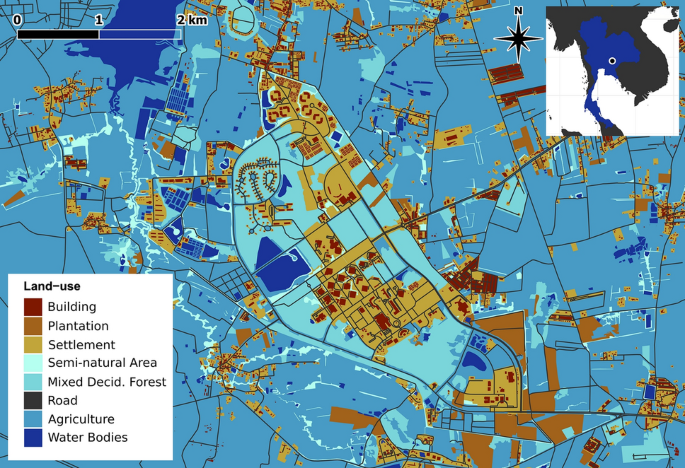This image depicts a detailed land-use map of a specific town, showcasing various land designations through a comprehensive color-coding system. It includes a scale bar that measures distances of 0 to 2 kilometers, with the first kilometer marked in black and the second in transparent. A cardinal direction cross with a star and the letter 'N' at the top signifies north. Additionally, a pictorial inset on the right provides a zoomed-out version of the main map for broader geographic context. 

In the bottom left corner, a key within a white rectangle defines the land-use classifications: buildings (maroon), plantations (brown), settlements (mustard yellow), semi-natural areas (light blue), mixed deciduous forests (medium blue), roads (gray), agriculture (dark blue), and water bodies (navy blue). Each of these categories is clearly represented on the map, with distinct color markers for easy identification. For example, settlements are concentrated in the center of the map, marked with light yellow areas interspersed with maroon dots indicating buildings. Surrounding these settlements are semi-natural areas, water bodies, and other land uses. Despite its detailed color coding, the map does not include street names or state identifiers, focusing solely on land-use patterns.